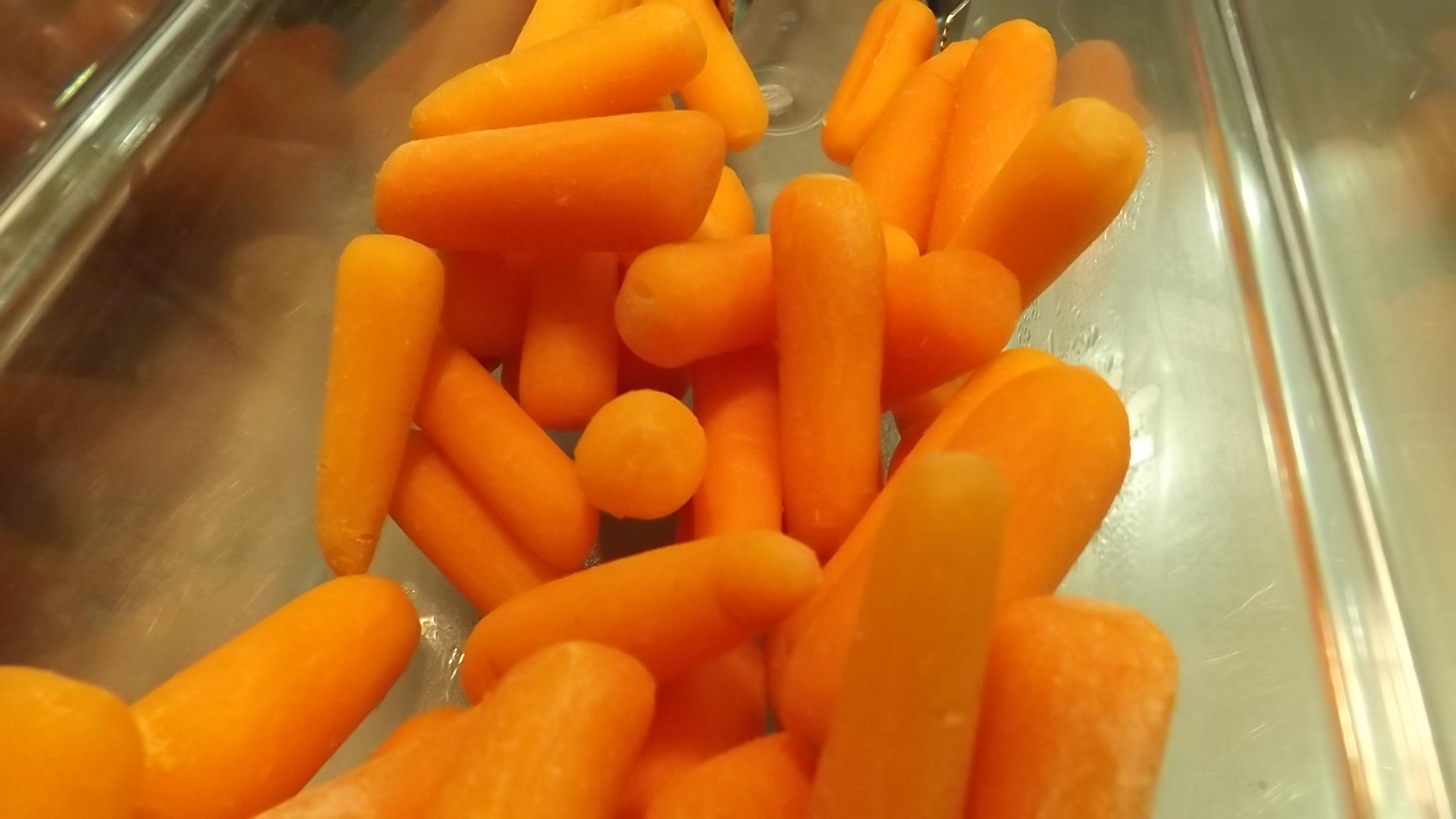The image prominently features a large, yellow plastic food storage container filled with peeled, baby orange carrots, each approximately 2 to 3 inches in length, totaling around 20 to 35 in various angles and shapes. The container is set against a white or yellow surface, and on the left side, a strong reflection of the carrots is visible due to the light source. The container has a noticeable ridge of raised plastic extending from top to bottom along the right edge, contributing to the structural design. In the back upper right corner, there is a dark shadowed area with an orange element peeking just below the top right corner, likely another carrot. The picture is overall simple, seemingly taken with a non-professional camera, as indicated by its dullness. Additionally, there appears to be a hand entering the frame from the bottom left, possibly interacting with the carrots.